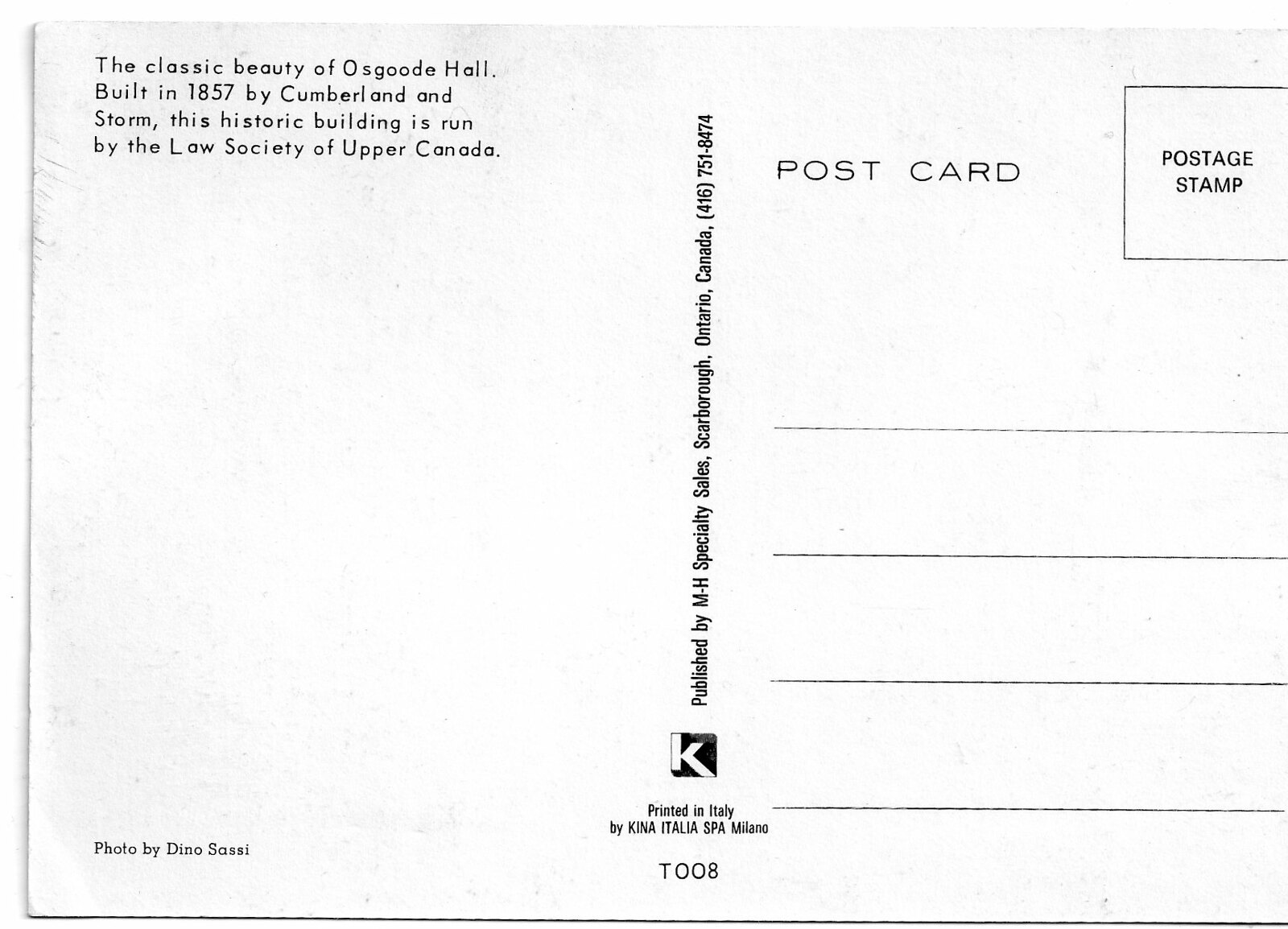The image is a scan of a slightly aged but blank vintage postcard. The postcard is entirely in black and white and showcases various informative details. In the top left corner, it reads "The classic beauty of Osgoode Hall, built in 1857 by Cumberland and Storm. This historic building is run by the Law Society of Upper Canada." Below this description, it states, "Photo by Dino Sassi." Centered vertically on the postcard, "Published by MH Specialty Sales, Scarborough, Ontario, Canada," is printed alongside a phone number. Below this text, there's a logo featuring a letter "K" against a black square, and the note "Printed in Italy by Kena Italia Spa Milano," accompanied by the code "T-008."

To the right, there are four blank lines designed for writing an address, with "POSTCARD" inscribed above them in all capital letters. In the top right corner of the postcard, a designated square is labeled "Postage Stamp." The postcard retains its typical simplicity, embodying a classic design with clearly marked sections for the sender's message and the recipient's address.